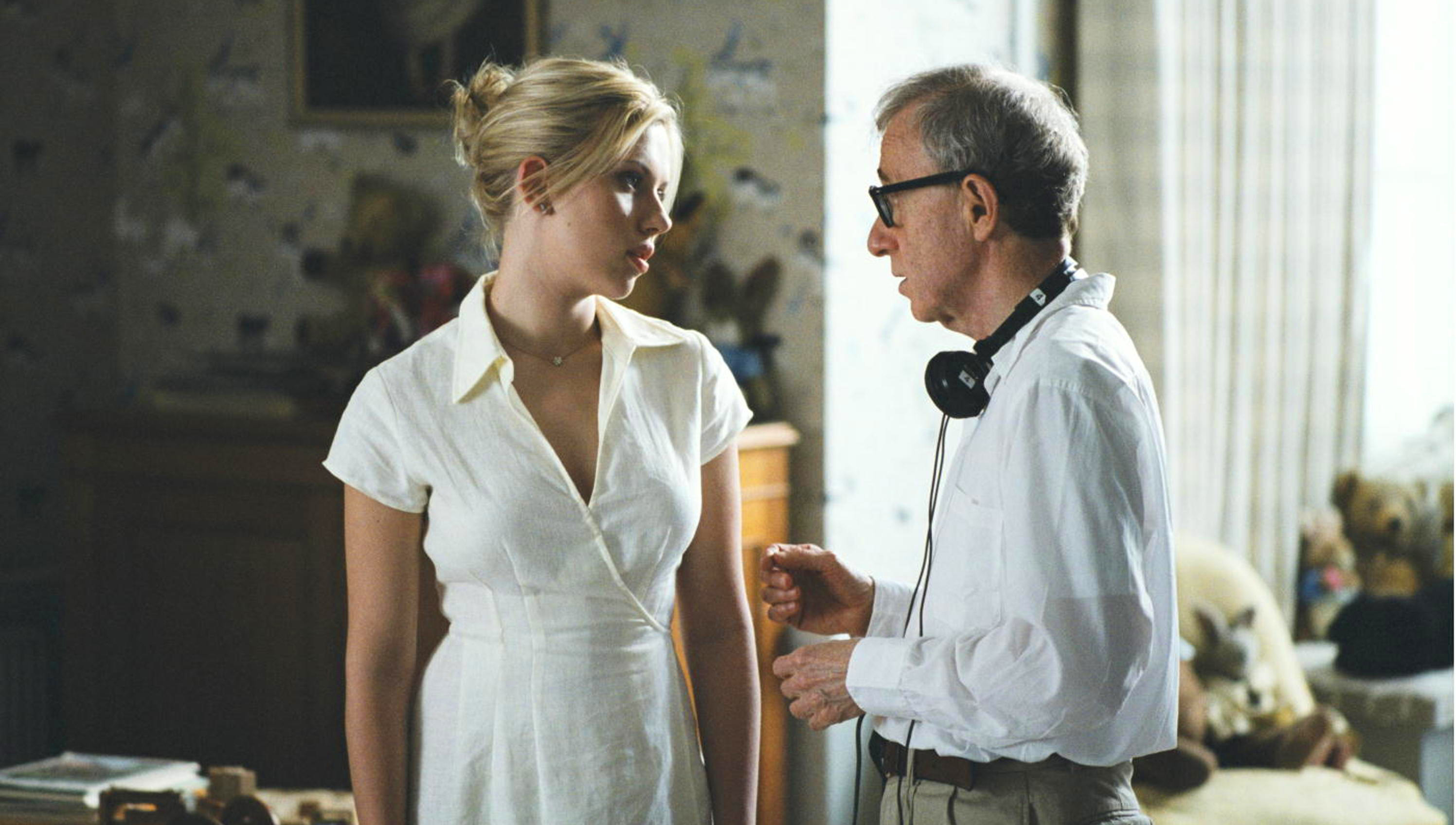In the image, a scene unfolds in a bedroom filled with subtle details. A woman with blonde hair, styled in an updo, stands to the left. She is clad in a white, short-sleeved blouse and wears a necklace, gazing intently at the man to her right with her mouth slightly open. The man, appearing somewhat older with short gray hair and black-rimmed glasses, faces the woman. He sports a pair of wired headphones draped around his neck, the cable hanging down over his chest. His attire includes a white, loose-fitting button-up shirt and gray pants secured with a brown belt. This intimate setting is decorated with light-colored curtains, a dresser, and a piece of artwork on the wall. Scattered stuffed animals, including a teddy bear, sit on a surface that could be a sofa or a cushion seat. Additionally, books are visible on a table, suggesting a thoughtful discussion or an instructive moment between the two.